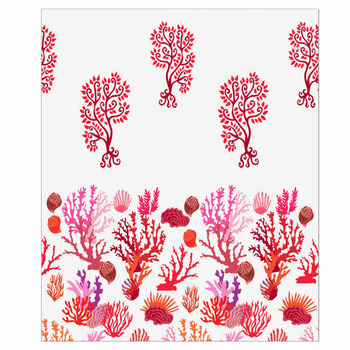This is a detailed digital artwork resembling a coral reef, set against a primarily white background. The bottom half of the image features a vibrant array of various corals and sea life depicted in shades of red, pink, violet, orange, and lilac. These elements, which include coral structures shaped like trees and seashells, seem to be assorted with slight changes in size, direction, and color, yet sharing a repetitive pattern. Above the corals, the scene transitions into a series of identical, slender, red coral or seaweed-like plants. These plants have a branching structure with leaves and appear to be strategically duplicated and flipped in different directions, creating a zigzag pattern across the top part of the image. The overall composition expertly combines these elements into a cohesive and artistic portrayal of underwater life, employing a mix of repetition and variation to evoke the rich diversity of a coral reef.